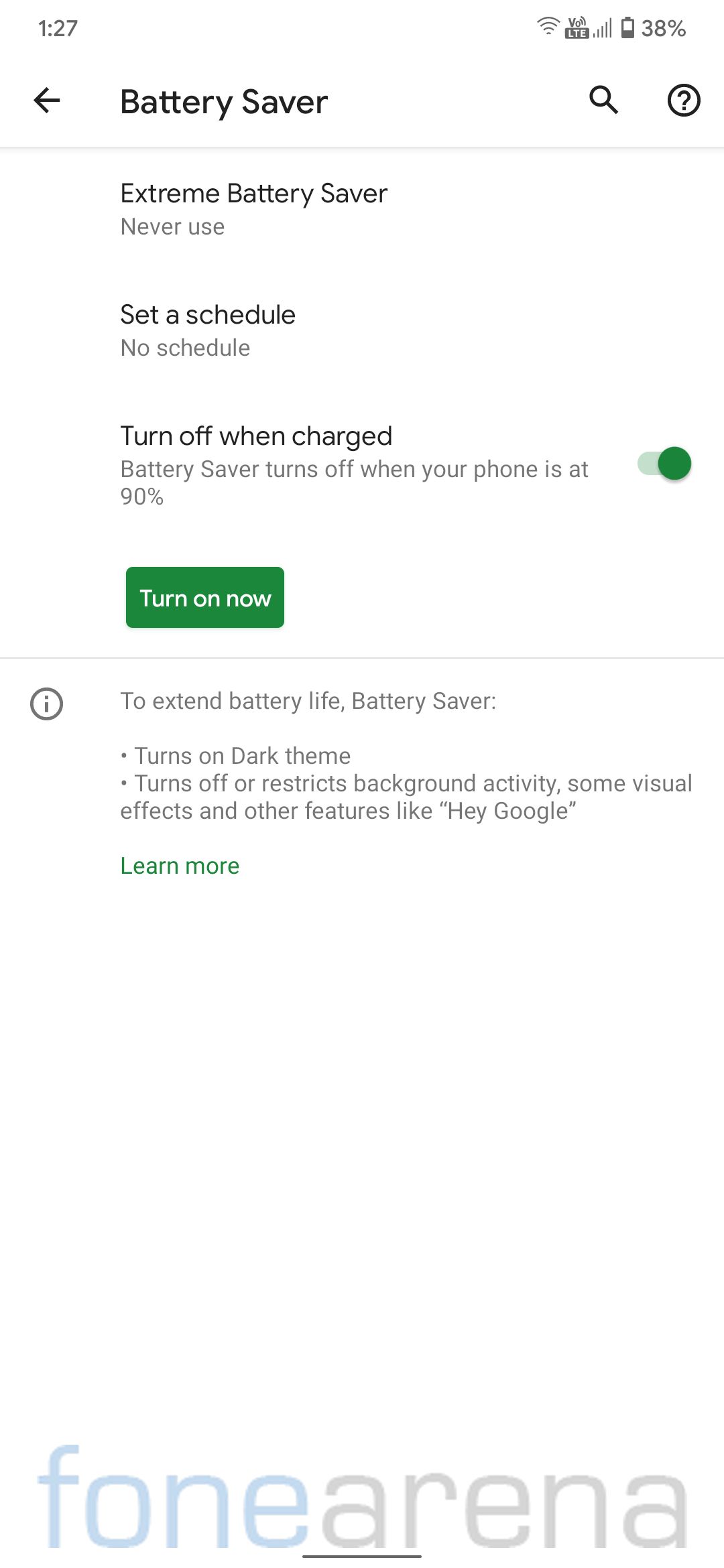A user navigates through the settings on an Android phone, specifically to the 'Battery' settings. They then access the 'Battery Saver' settings menu. Within this menu, several options are displayed: the 'Extreme Battery Saver' mode is set to 'Never Use', there is no schedule set for the battery saver, and the 'Turn off when charged' toggle is enabled, meaning the battery saver turns off automatically when the battery reaches 90% charge. There is also a button labeled 'Turn on now' which appears active, despite the default setting showing the battery saver as off. The description clarifies that enabling the Battery Saver mode activates features such as a dark theme, restricted background activity, and the disabling of certain visual effects and functionalities like 'Hey, Google,' thereby optimizing battery life.